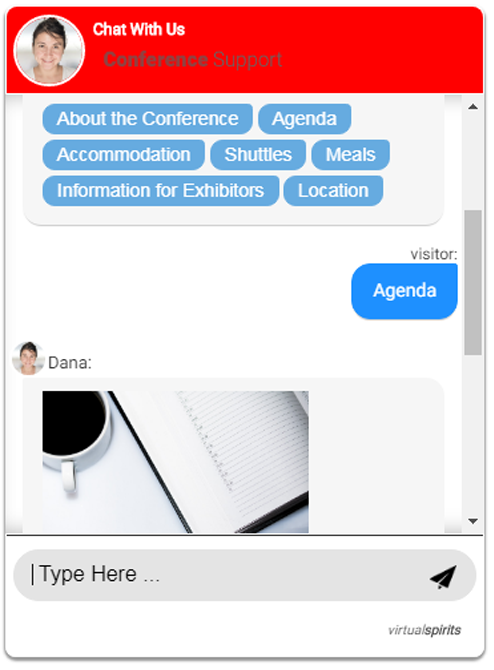This image depicts a help desk support interface designed for a conference. At the top of the screen, it prominently displays the message "Chat with us" in white letters. Directly below that, the text "Conference Support" is visible, with the word "Conference" in bold dark blue font and "Support" in regular characters of the same color.

On the left side of the interface, there is an icon of a smiling woman who appears to be in her late 20s to early 30s. She has black hair and is wearing a white top, set against a blue and white background. Below this icon, there are several interactive buttons organized into three lines. The first line includes buttons labeled "About the Conference" and "Agenda". The second line features "Accommodation," "Shuttles," and "Meals". The third line contains buttons for "Information for Exhibitors" and "Location".

Underneath this section is a large white area containing the text "Visitor:" followed by a blue button labeled "Agenda". Adjacent to this, the same image of the support person, named Dana, appears as seen in the upper left corner. Accompanying the image is a date book and a cup of black coffee. Below this, there is a text input field with the placeholder text "Type here..." and a send button depicted as a folded paper airplane.

Finally, at the bottom right corner of the interface, the branding "Virtual Spirits" is displayed.